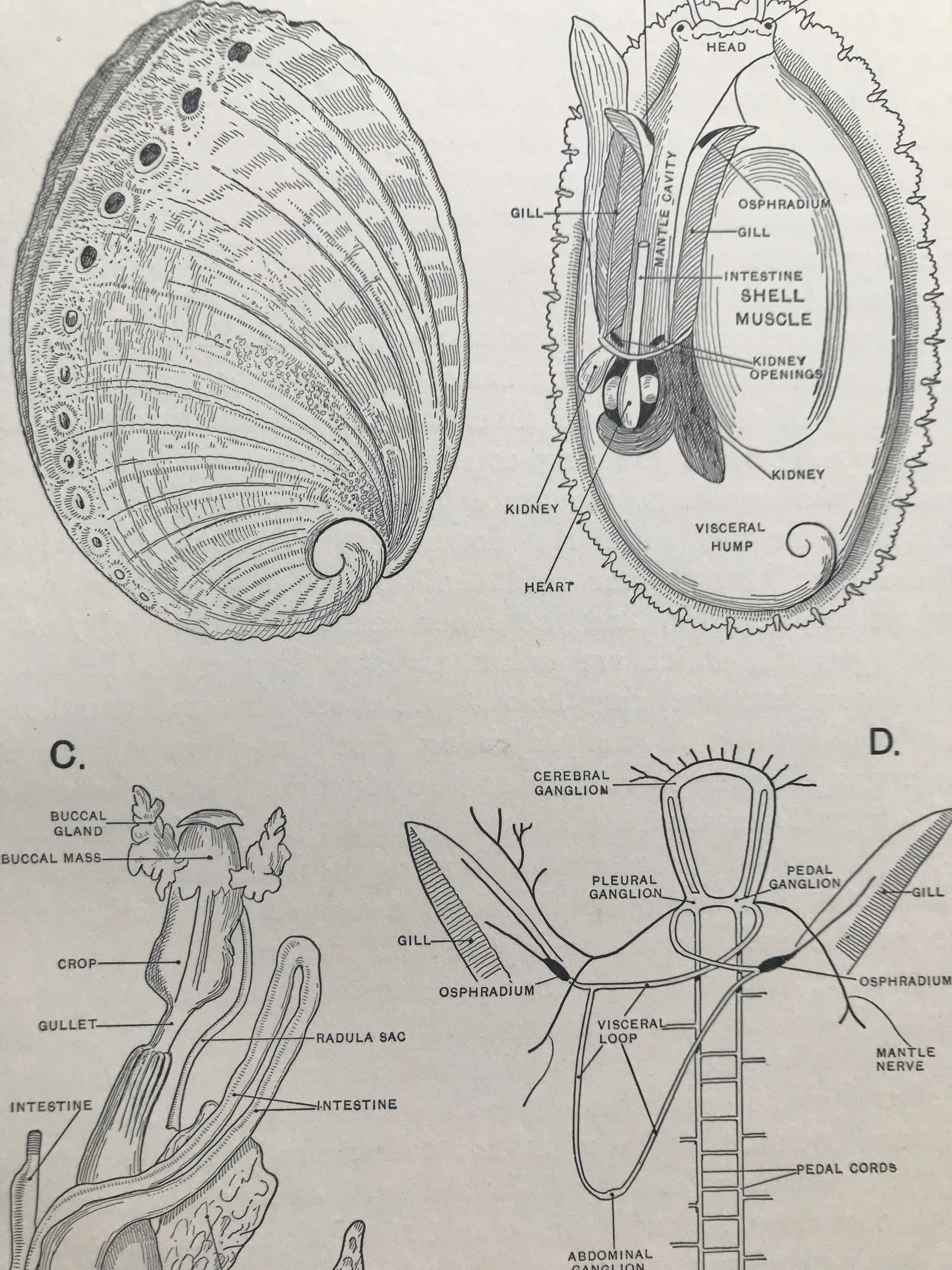The image is a black-and-white illustration from a science textbook depicting the anatomy of a mollusk, specifically a snail. The top left section shows a whole shell as viewed from the outside, while the top right features a detailed cross-section of the snail inside the shell, labeling parts such as the head, gill, intestine, shell muscle, kidney opening, visceral hump, heart, and kidney. The lower left section, labeled C, provides a detailed view of the intestinal system, including the buccal gland, buccal mass, crop, gullet, intestine, radula, sac, and intestine. The lower right section, labeled D, contains a detailed view that possibly includes the head and nervous system, indicating structures such as the visceral loop, gill, pleural ganglion, cerebral ganglion, gill, and mantle nerve. Each section comprehensively labels various anatomical features to offer a detailed insight into the snail's structure.